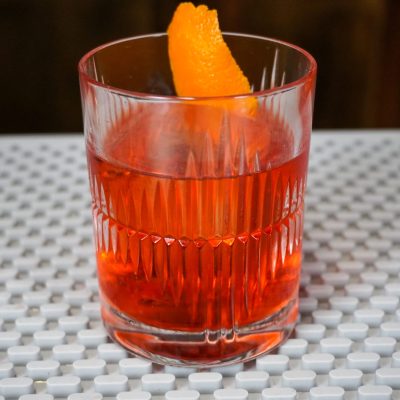This up-close image showcases an intricately detailed cocktail in a lead crystal glass, accentuated by its variegated edges. The apricot rose-colored liquid fills the glass about three-quarters full, with a uniquely carved lemon peel garnish that features indentations, creating three distinct points. The glass rests on a white mat composed of an arrangement of interconnected discs, raising it slightly from the surface. The background is a stark black, contrasting with the bright, inviting colors of the drink and mat below.